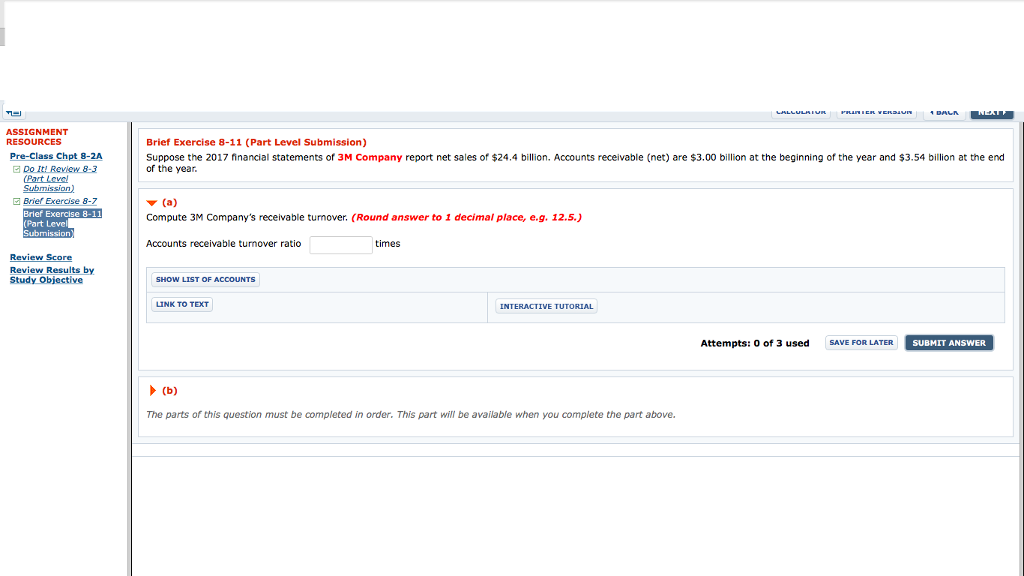The image features a light blue background. At the top, a light blue line runs horizontally from about half an inch down the left side, extending across the top edge with a thin black line embedded within it. Beneath the top line, there is a small blue box containing some very tiny text. 

On the left side, bold red text reads "Assignment Resources," followed by blue text that says "Pre-Class Chat 826," beneath which are several bullet points, with one of them highlighted. To the right of this section, a thick blue line separates it from a white box with red text reading "Brief Essentials 911," alongside text indicating "Part Level Submission" and additional printed details.

Further to the right, another white box contains a downward-pointing red arrow next to the letter "A." Below this, red text and more blue text are visible, accompanied by two blue boxes followed by a third blue box on the far right side. Another white box indicates "Attempts 0 of 3," and includes a very small blue button labeled "Save for later" alongside a larger blue button that says "Return or submit answer."

Finally, another white box features a right-pointing red arrow next to the letter "B." A blue line is present within this section, and the overall layout concludes with an additional blue line on the right side of the image.